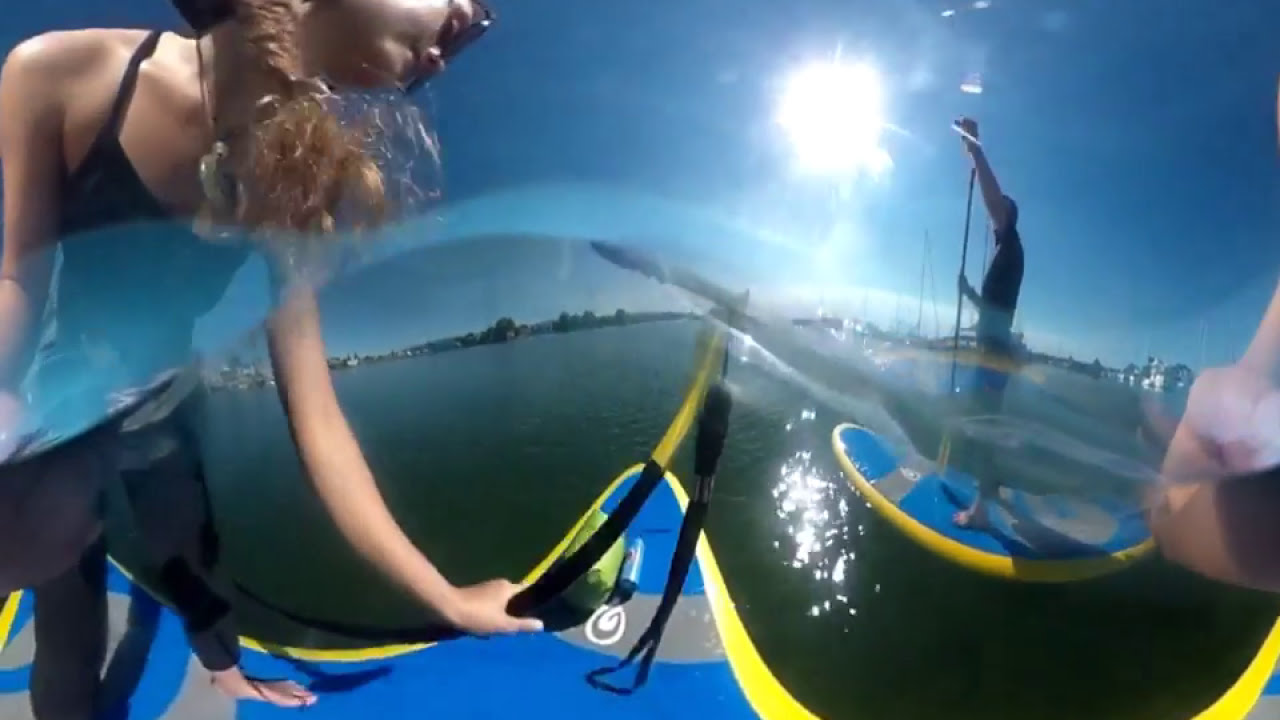In this somewhat distorted 3D image, we see two individuals paddleboarding on a body of smooth water. To the left stands a light-skinned young woman with long, strawberry-blonde hair tumbling over her shoulder. She is wearing white sunglasses, a black spaghetti-strap tank top, and black pants, possibly a wetsuit. She appears to have a jacket tied around her waist and is barefoot. Her attention is directed downward towards her paddleboard, and she holds a curved paddle from which a black strap hangs.

To the right of the picture, there is a male figure on a similar blue paddleboard with yellow trim. He is dressed in black clothing and holding an oar with one hand stretched upward and the other midway down the pole. The intense, bright sun casts a fair amount of glare and shines just to his left. The backdrop features a clear blue sky with a visible skyline of buildings and masts of sailboats in the distance, and some land can be seen off to the right. The sun is high, casting shadows to the right and contributing to the image's hazy atmosphere.